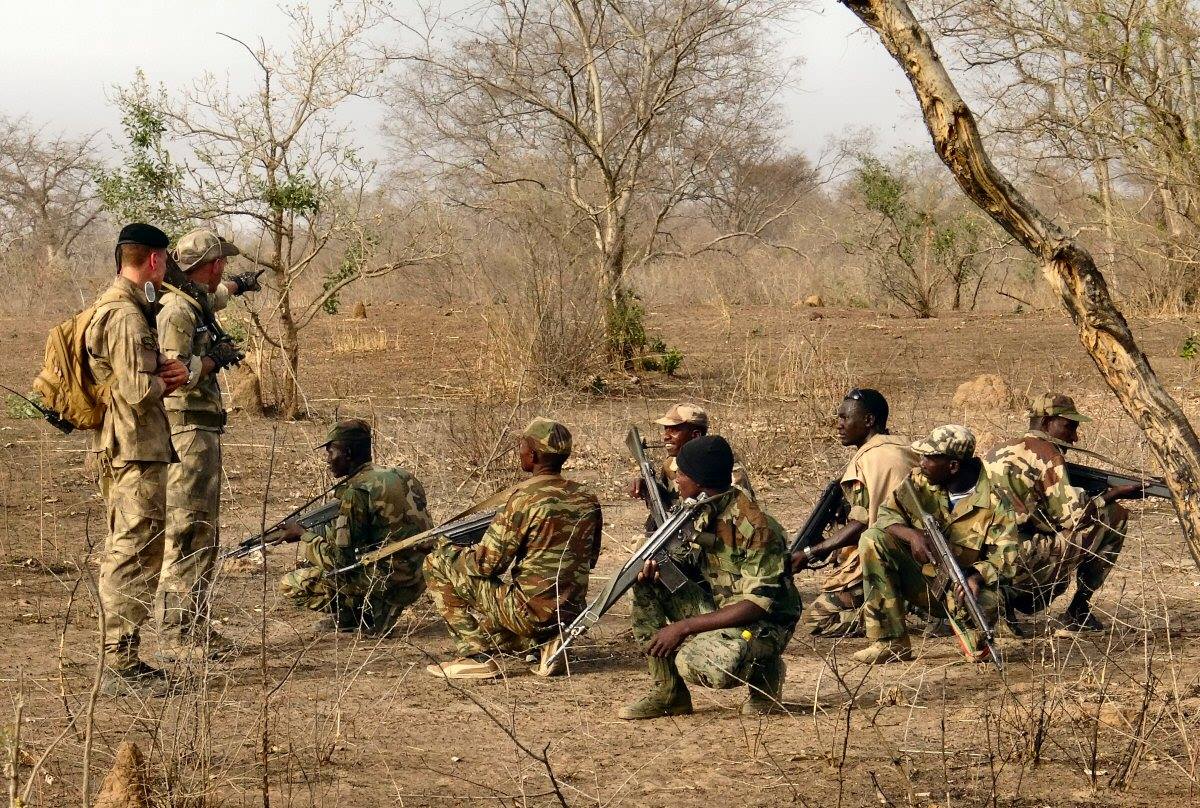In the image, a group of African soldiers donning green and tan camouflage uniforms are kneeling or crouching on dry, sparsely vegetated terrain, likely in a jungle or desert area in Africa. The scene is dominated by leafless trees, though a few have some sparse green foliage. Each soldier holds an assault rifle, and some wear hats while others do not. All the kneeling soldiers are black, and they appear attentive to two standing figures who seem to be leading or instructing them. One of these standing men, who is white, wears a camouflaged hat and points into the distance, possibly at an animal. The other standing figure, who has short black hair, wears a tan backpack and different shades of camouflage, and observes the scene. The overall atmosphere suggests a military training or briefing session in a challenging, dry environment.